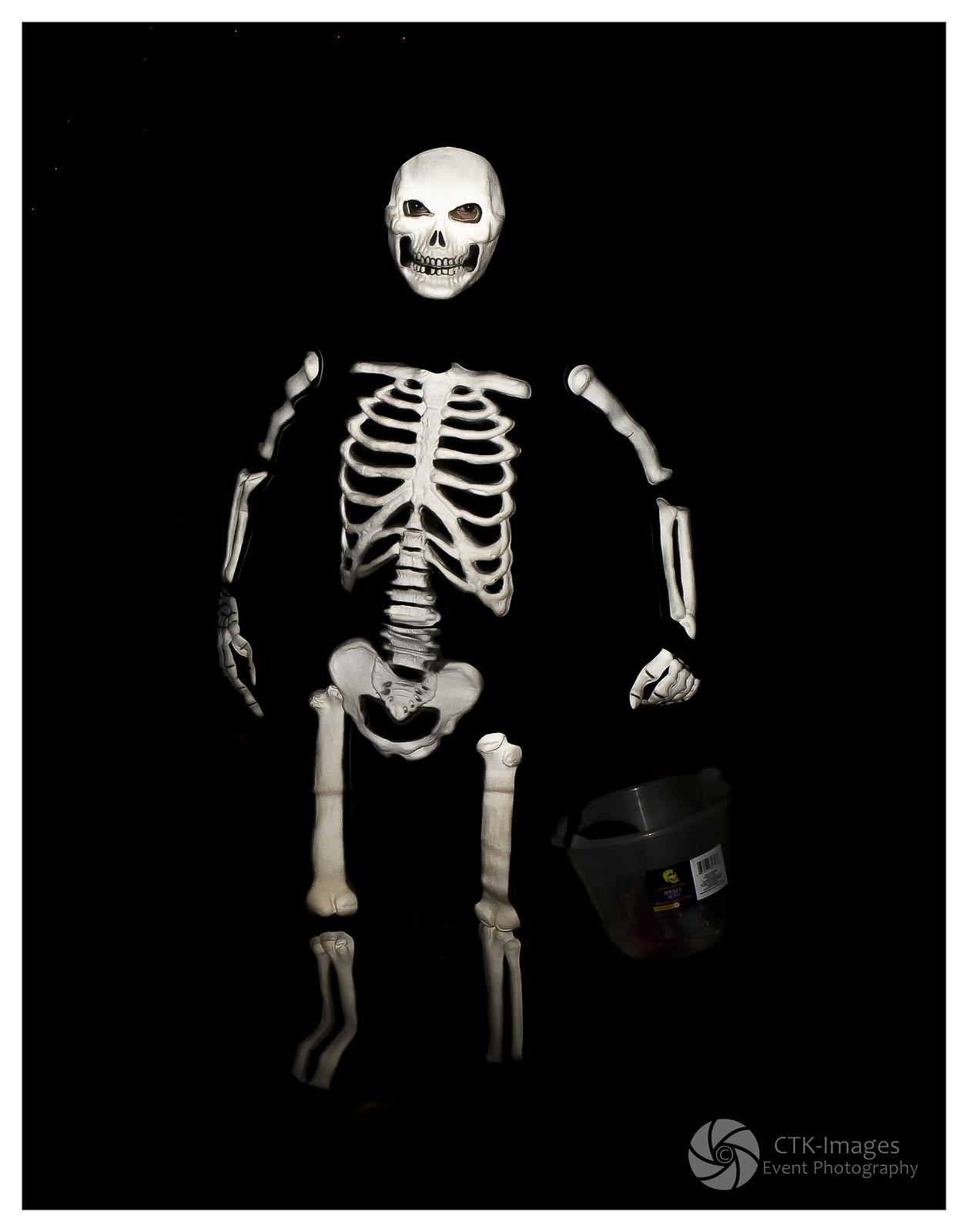This black-and-white photograph captures a person in a full-body skeleton costume set against a completely black background. The costume features detailed skeletal bones, including gloves and a skull-shaped face mask, with the skull appearing to float in mid-air due to the lack of visible neck or shoulder connection. The person's eyes are visible through the mask, highlighting the human presence behind the eerie facade. In their left hand, they hold a dark, possibly metal, bucket or pail, presumably for collecting candy on Halloween. The image bears a watermark in the lower right-hand corner, displaying a logo resembling a camera shutter beside the text "CTK Images Event Photography." Overall, the stark contrast between the white bones and the black backdrop emphasizes the haunting effect of the costume.